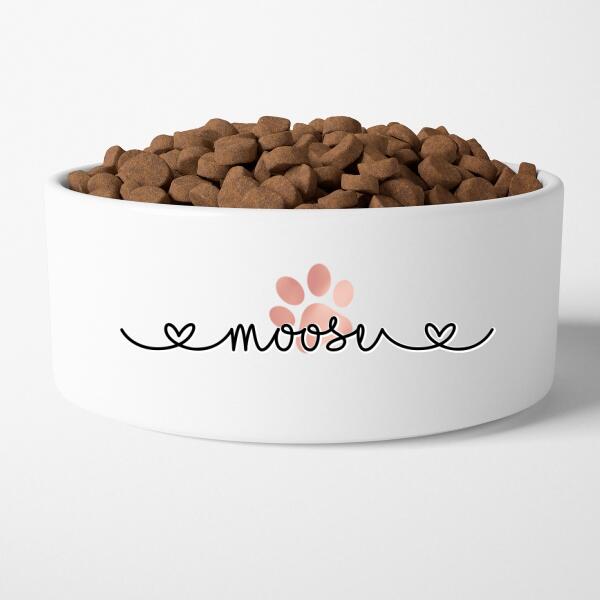The image is a color photograph of a white ceramic bowl filled to the brim with small, brown kibble, slightly overflowing. The bowl, set against a plain white background, features a pink paw print and the name "mooser" written in lowercase cursive script, starting and ending with a heart motif. This detailed design suggests that the bowl belongs to a pet named Mooser, whether a dog or cat.